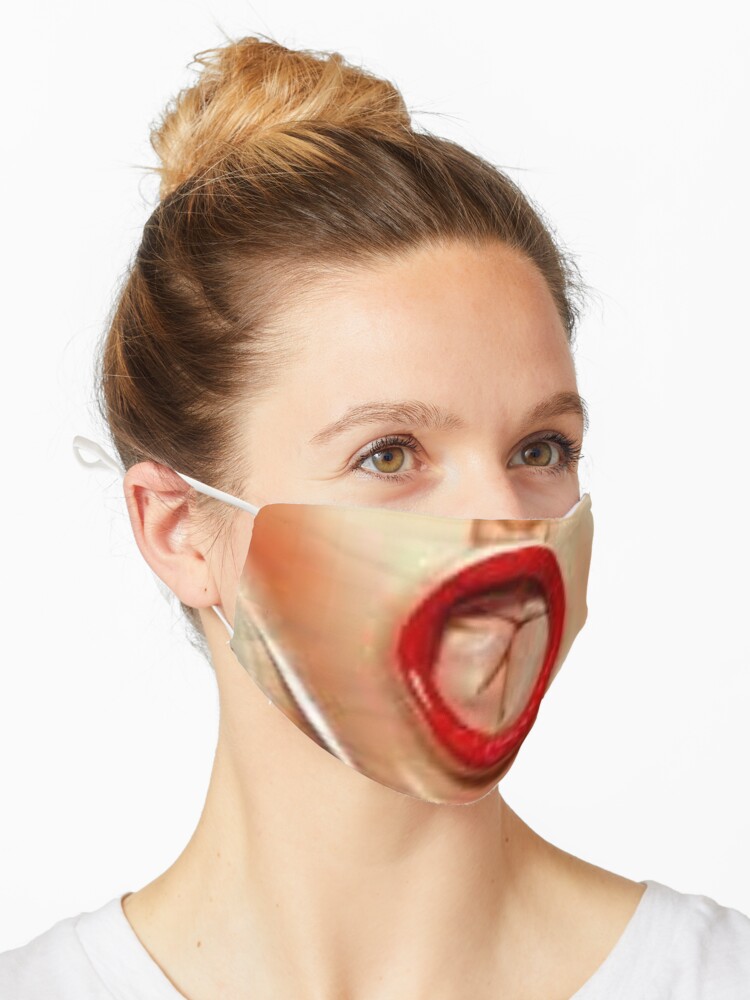In the image, there is a headshot of a woman with dark brown hair styled in a blondish, yellowish bun. She has greenish-brown eyes and is wearing a white t-shirt. The background is completely white. Her face is partially covered by a peculiar face mask. The mask is secured with white strings behind her ears and is designed to mimic a wide-open human mouth with exaggerated red lips, reminiscent of a gag gift or a humorous accessory possibly meant for a Halloween costume. The mask's surface is shaded beige to resemble skin, and the mouth depicted on it has an unusual circular shape, giving the overall impression of a playful and comical appearance.